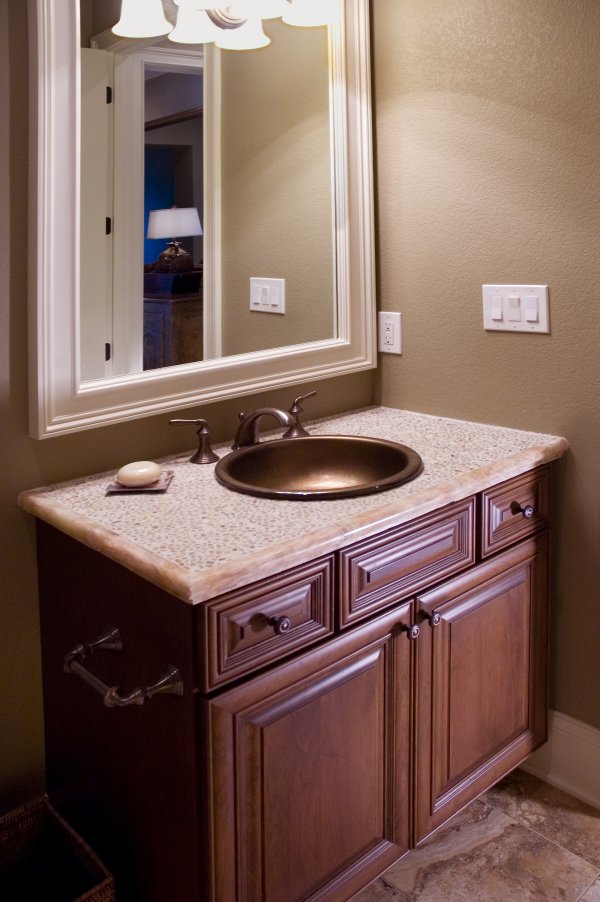This photograph captures a cozy corner of a bathroom featuring a stylish vanity and sink area. The walls are painted in a warm light brown or dark tan, providing a serene backdrop for the furnishings. The vanity, made from dark-colored wood, has a striking pebble stone countertop in shades of white and tan. A round, brown-bronze sink and matching bronze faucet set add a touch of elegance. To the left of the sink, a round bar of white soap rests atop a square dish. Above the sink hangs a tan-framed mirror, reflecting a glimpse into an adjoining room. In this reflection, you can see a doorway leading to a room with a round brown lamp with a white lampshade sitting atop a table. Next to the mirror, on the right wall, there is a white outlet and a light switch panel with three switches. The flooring is a modern brownish tile that complements the bathroom's color scheme. On the left side of the vanity, there’s a towel holder displaying a small hand towel.